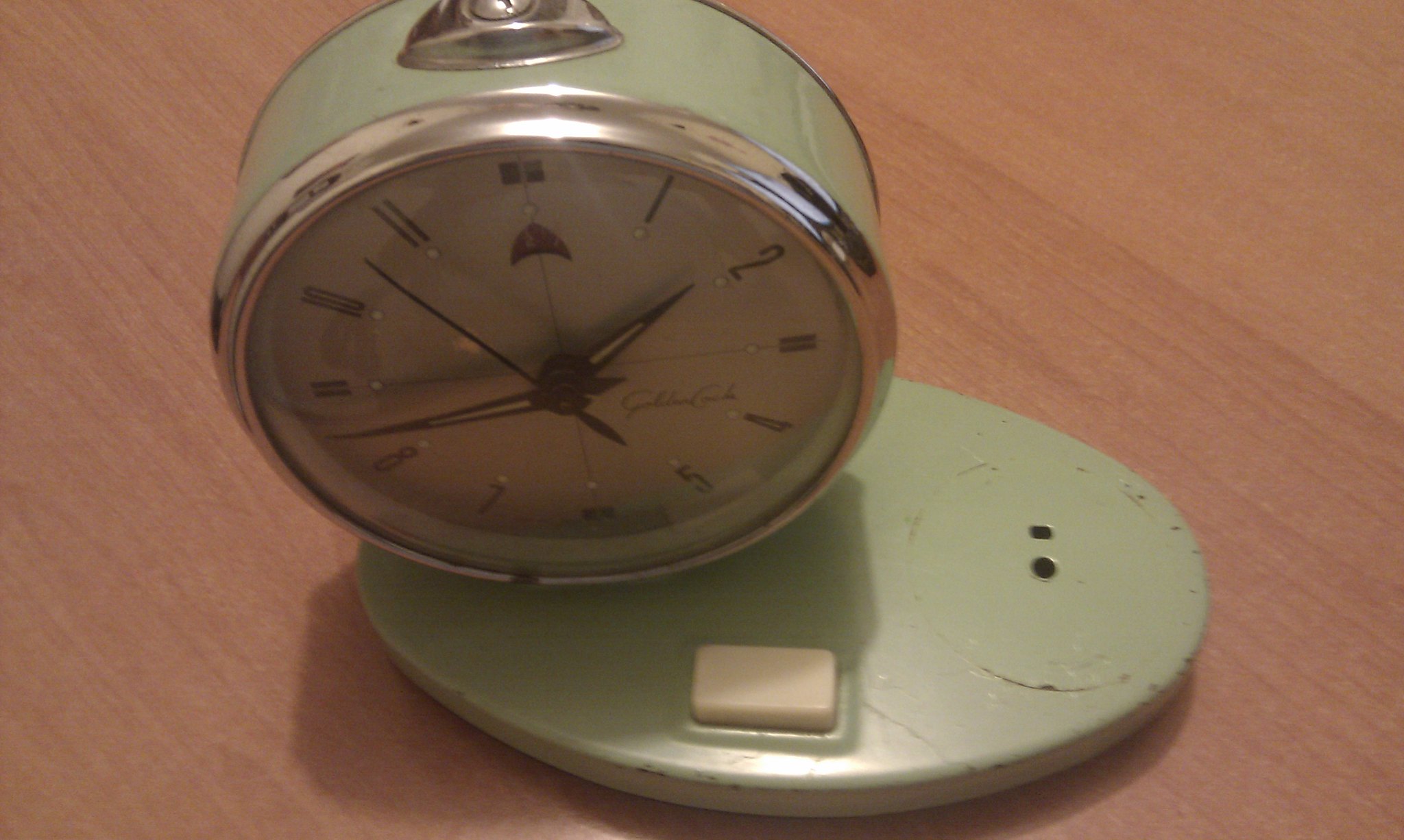This photograph features a vintage-style, retro clock with a white and green body. The clock has a round face with a chrome rim and showcases black, vintage-style numerals against a white background. Its black hands are clearly visible. A white button is located on the green base of the clock, and a silver metallic object sits atop it. The clock rests on a blonde wood surface, emphasizing the visible wood grain. The image quality is somewhat grainy, and the clock casts a shadow on the table. The clock appears slightly dirty, with noticeable brown dirt or chipped paint on its surface.